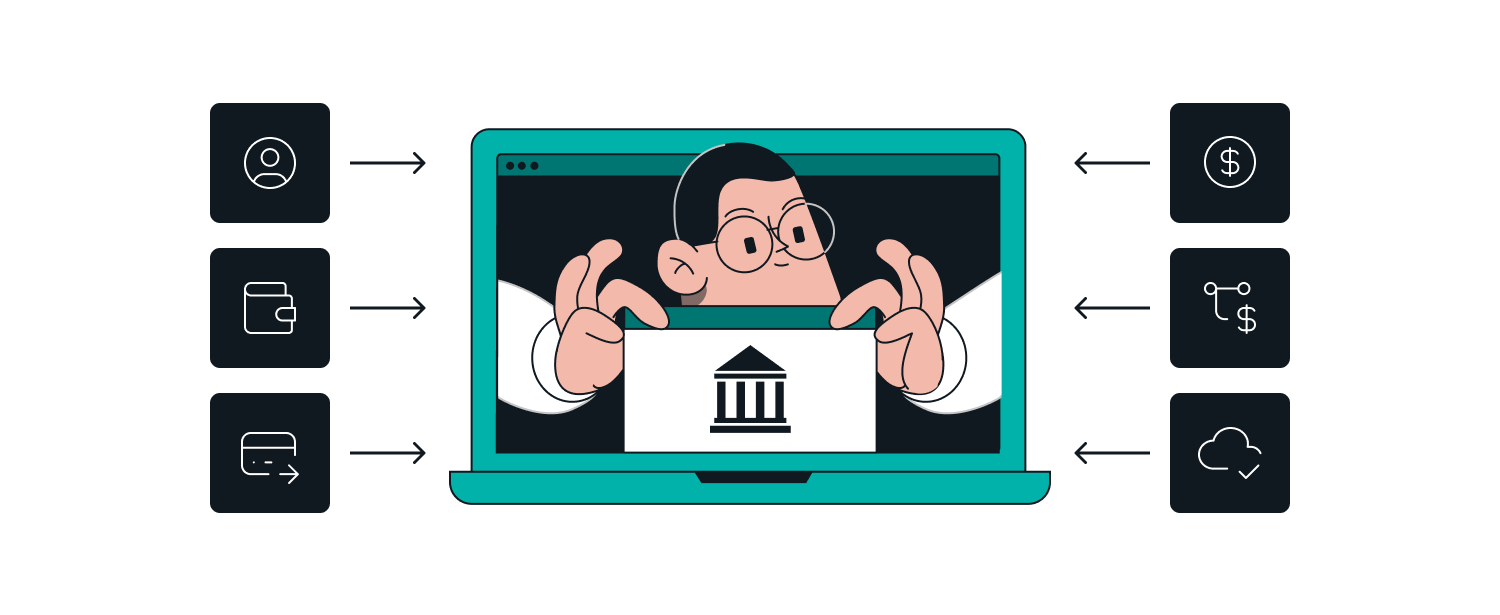The image is an infographic illustration featuring a prominent, open teal-colored laptop at the center. Displayed on the laptop screen is a cartoon man with circular glasses, dark short hair, and white sleeves, though his elbows are cut off by the edges of the screen. The man, who almost appears monkey-like due to his features, is holding a card with a black image of a columned bank building with a pointy roof on a white background, and a teal border similar to the laptop.

Surrounding the laptop are six black boxes, three on each side, with white icons representing different functionalities. On the left side, from top to bottom, are icons of a profile outline, a wallet, and a key or passkey outline. On the right side, the boxes showcase a dollar sign within a circle, a symbol of shared money with smaller dollar signs and lines, and a cloud with a checkmark indicating cloud saves. Black arrows point inward from the boxes towards the central laptop, emphasizing that these functionalities are part of the laptop's features.